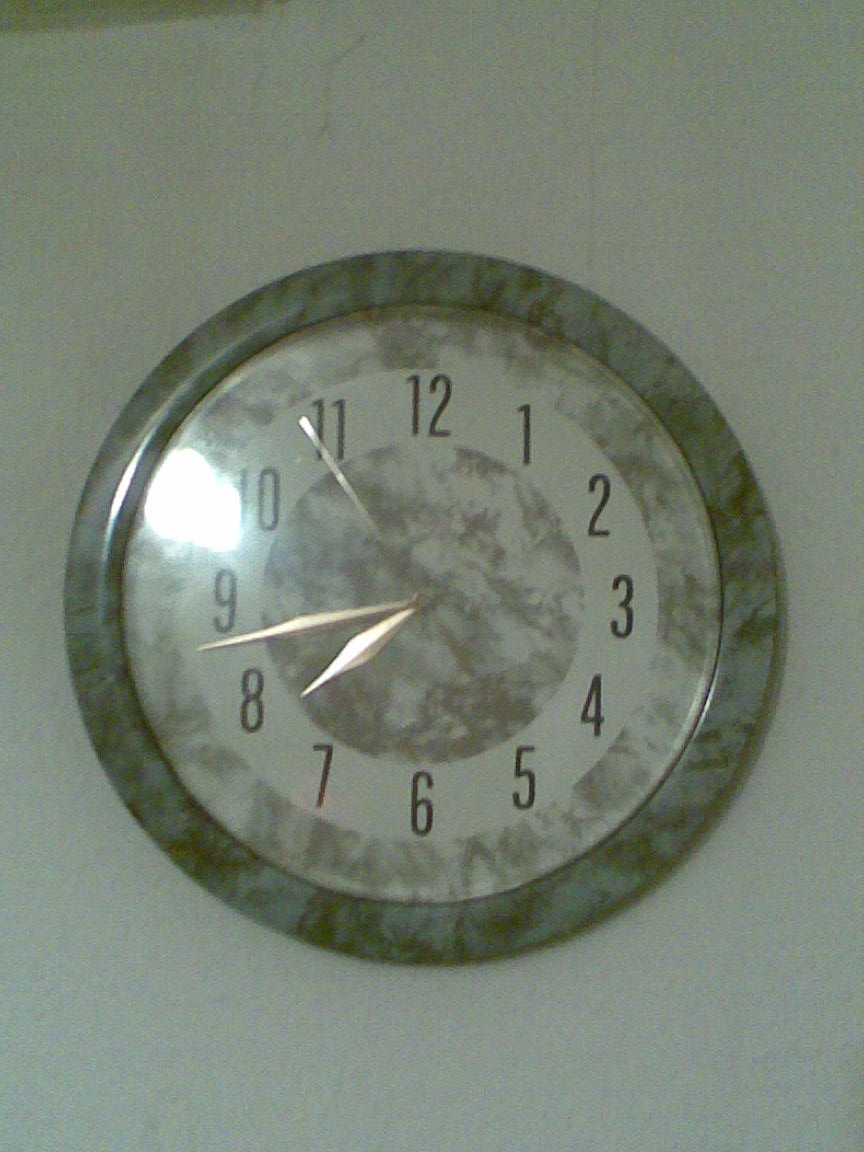The image depicts a wall clock mounted on a grayish-white wall. The clock features a striking green marble-patterned border interspersed with black accents. The clock face mirrors the design of the border but in a slightly lighter shade of green combined with white. At the edge of the face, there is a white circular ring within which the black numbers are displayed. The inner section of the clock face retains the green marble pattern. The clock's hands, appearing to be either silver or gold, are positioned to indicate the time is approximately 7:43.